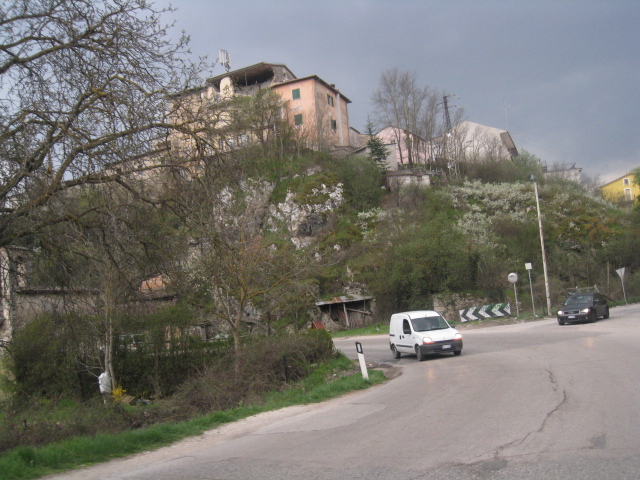The photograph captures an atmospheric street scene in a seemingly old European town. In the lower third of the image, a curving gray road meanders into view, with a white utility vehicle approaching a black car stationed at an intersection. To the left of the road, thick foliage frames what appears to be a building, possibly a house or shop, partially obscured by bare trees and a singular white leafy tree by a porch. Alongside the road, patches of gray-green grass and a white post marked "Y" are noticeable. Above the scene, a rocky hill rises, crowned with a large, possibly 1930s-40s pink building with a dark roof and an antenna, giving it an abandoned and slightly derelict appearance. This building, possibly an old manor or university structure, is accompanied by a white building with a similar rundown aesthetic. Scattered among the hill's foliage are the tops of other buildings, including a partially visible yellow structure further down the road. Amidst this quaint yet decaying townscape, the sky stands clear blue, sprinkled with minimal cloud cover, enhancing the nostalgic charm of the setting.